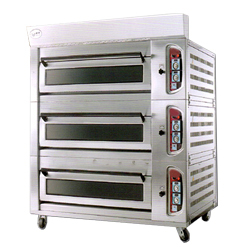This commercial pizza convection oven features three sleek, chrome silver oven doors, each with a long black handle for easy downward pulling, allowing access to its narrow openings—sized perfectly for pizzas or trays of rolls. Each oven compartment is topped with a dark window, ensuring visibility of the contents. Flanking each door on the right are control panels boasting temperature and fan speed settings, enabling precise cooking control. The unit stands on four casters, providing mobility, although only three are visible in this mostly front-facing shot with a partial side view. The oven's top is accentuated with a white border, all set against a pristine white background, suggesting it's primed for catalog or advertisement display.